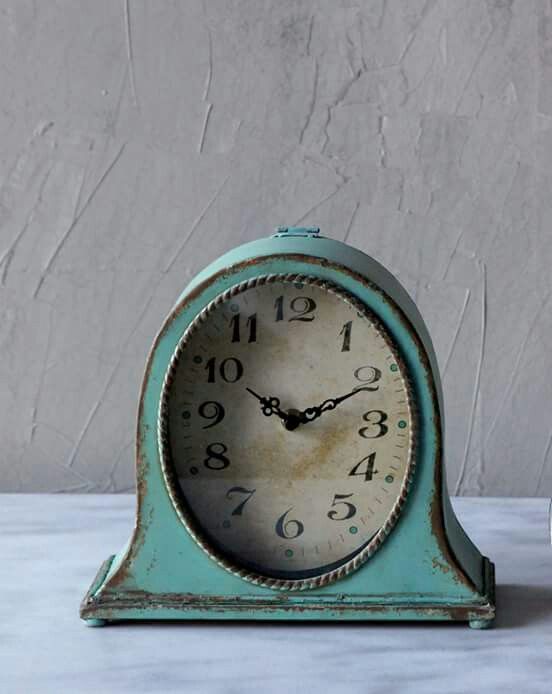This is a color photograph of a decorative, vintage clock sitting atop a weathered white surface, likely a dresser or shelf. The clock features a turquoise blue casing with areas of intentional wear, giving it a shabby chic or antique appearance. The oblong-shaped clock has an arched or oval top and a broader base. The face of the clock is framed by a braided metal decoration and sports an ivory or ecru background, possibly with a browned texture in the middle. The numbers 1 through 12 are displayed in an old-fashioned black font, and the clock hands indicate the time as 10 minutes after 10. Behind the clock, the wall is finished in thickly textured white plaster, showcasing distinct trowel markings. The photograph is brightly lit by sunlight peeking in from the left-hand side, suggesting it is daytime. There are no people, animals, or any other objects in the image, which focuses solely on the clock and its setting.